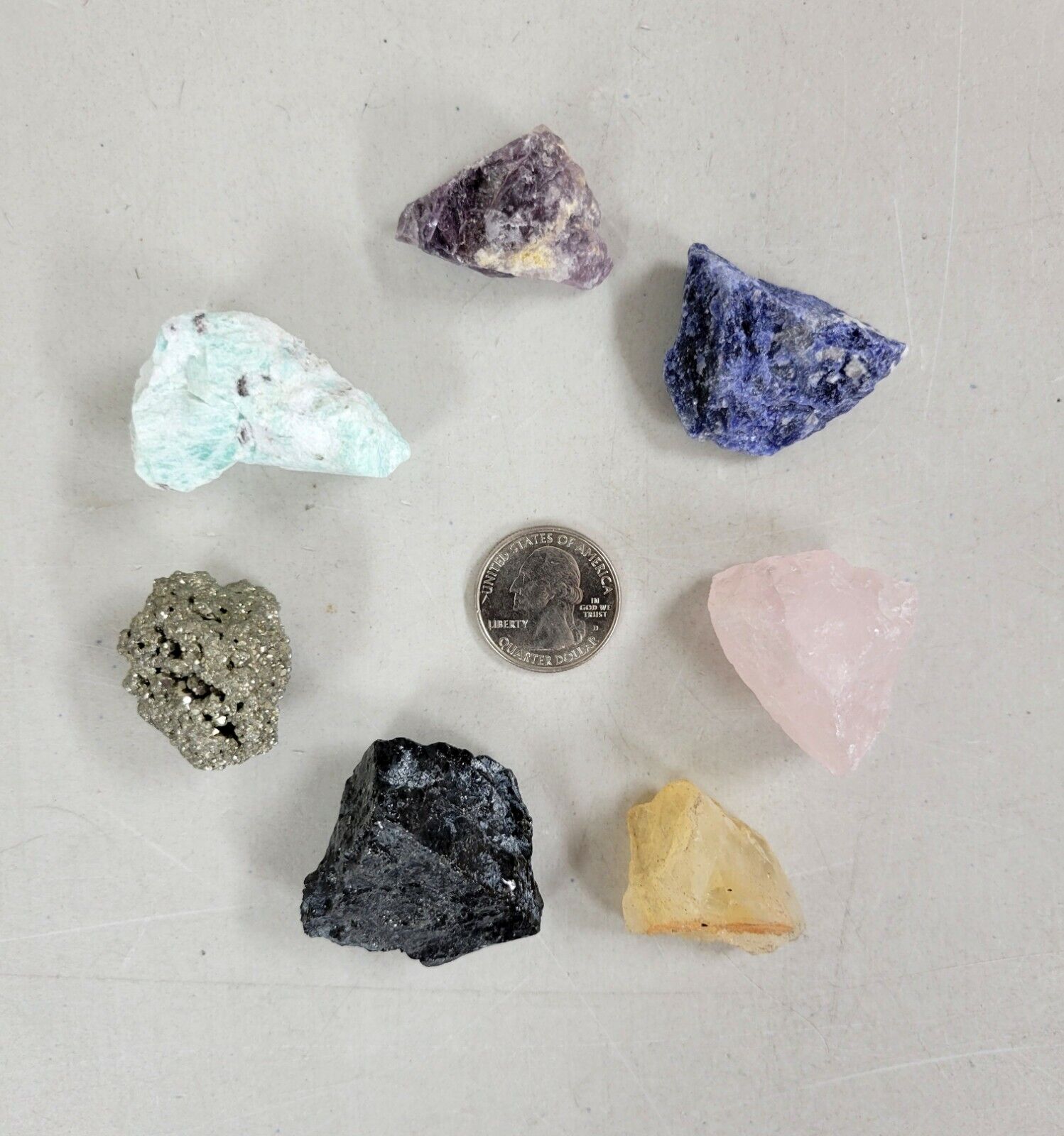The photograph displays a rockhound's collection meticulously arranged on a white sheet of paper. At the center is a shiny quarter featuring the head of George Washington with the inscription "United States of America" and "Quarter Dollar" for size reference. Surrounding the quarter are seven diverse mineral specimens, artfully positioned in a clockwise circle. At the top is a purple crystal, possibly amethyst. Moving clockwise, the next specimen is blue with white veins, likely lapis lazuli. The third stone is translucent pink, resembling rose quartz. Positioned next is a pale amber stone, which may be a type of agate. Following this is a shiny black piece, possibly a chunk of jet. Next is a silvery gold sparkling stone, identified as iron pyrite. Finally, the last specimen is bluish-white, potentially calcite or a similar mineral. The collection is evenly lit from above, enhancing the natural beauty of the stones against the white background.